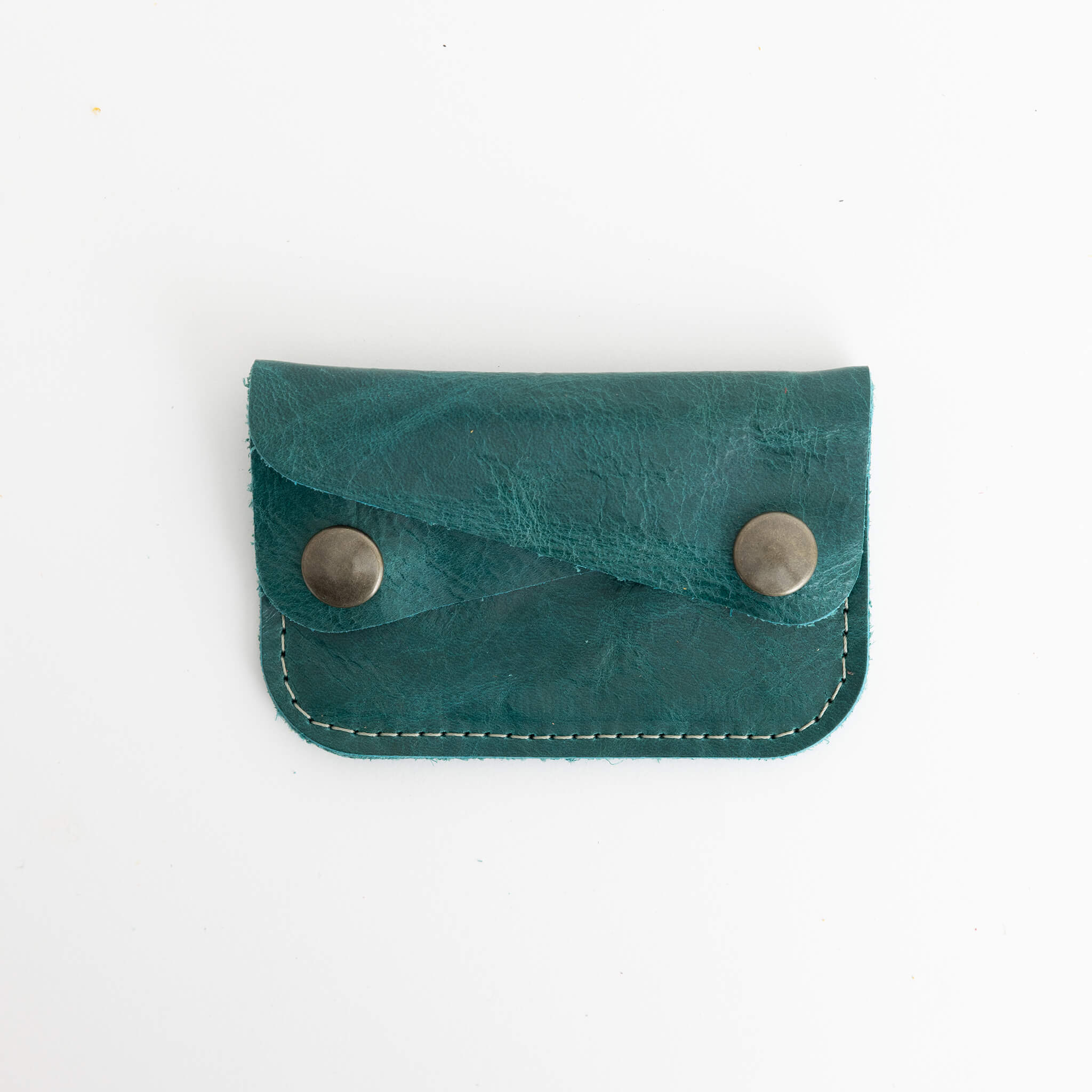In the center of the photograph set against an off-white background, there is a small, rectangular change purse resembling a leather or suede material with a rich, emerald-green hue. The surface of the purse showcases a refined grain texture, and it is accentuated by neat, tan-colored stitching along the bottom edge. The purse features two silver-colored snap buttons, one on each side of the top flap, which help secure it closed. The overall shape is slightly U-shaped with curved bottom edges. The image focuses solely on this compact and stylish accessory, devoid of any text, people, or additional objects, highlighting its design and functionality.